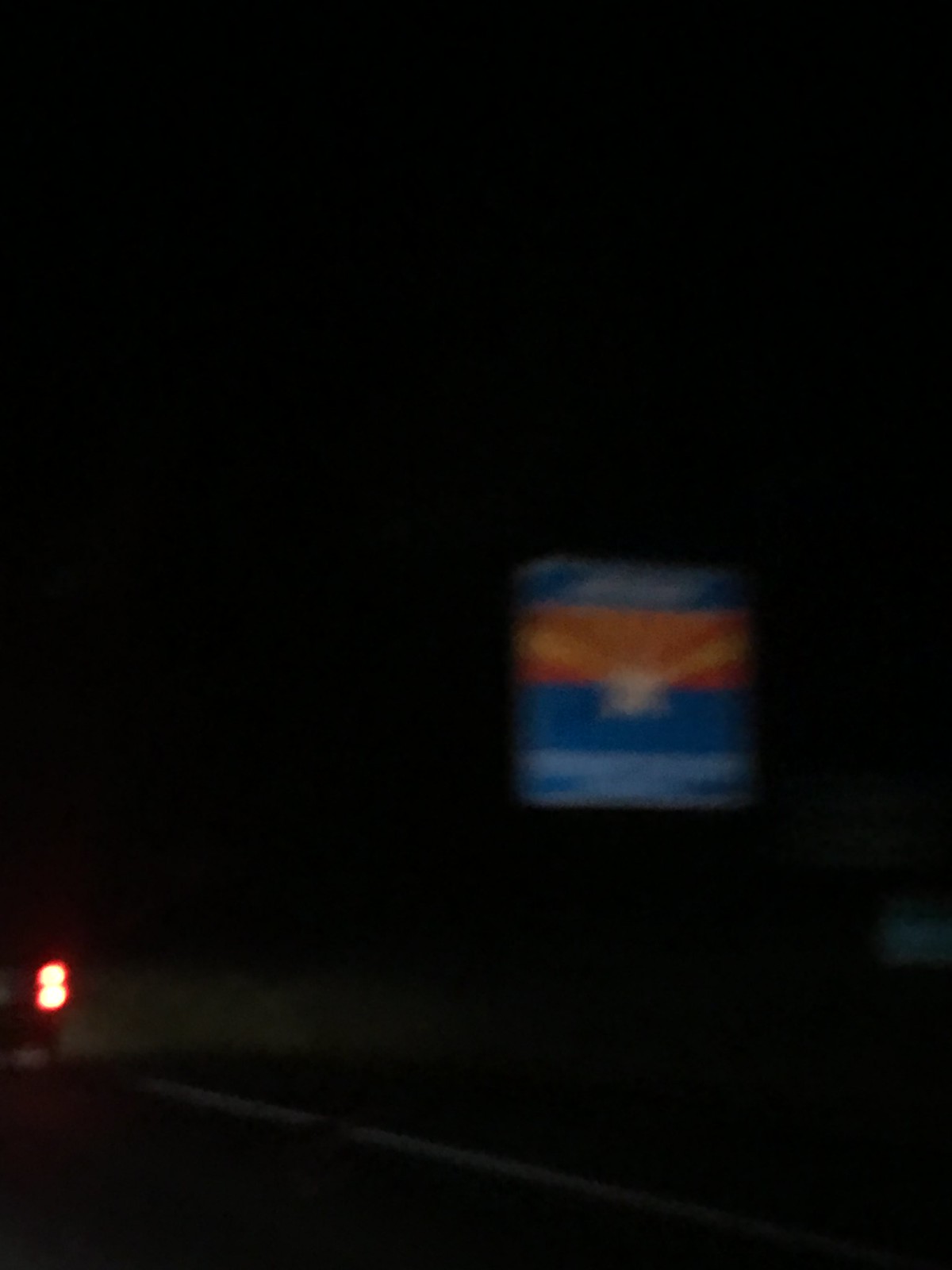The image predominantly features a dark, almost entirely black background, accented by points of light and color. In the lower left corner, there is a bright spot that appears to be a single light source, likely from a tiny LED, but due to the camera’s movement during capture, it manifests as two small, blurred beads of light. In the upper center right section of the image, there's the display of a digital device—possibly a cell phone, laptop, or television—imbued with a vintage aesthetic. This screen is also affected by the camera’s motion, creating a smeared effect with hues of orange, blue, and aqua blue against the black backdrop. The dynamic blur and trailing lights emphasize the photograph’s energetic, yet nostalgic ambiance, as if capturing a fleeting moment in a low-lit environment.